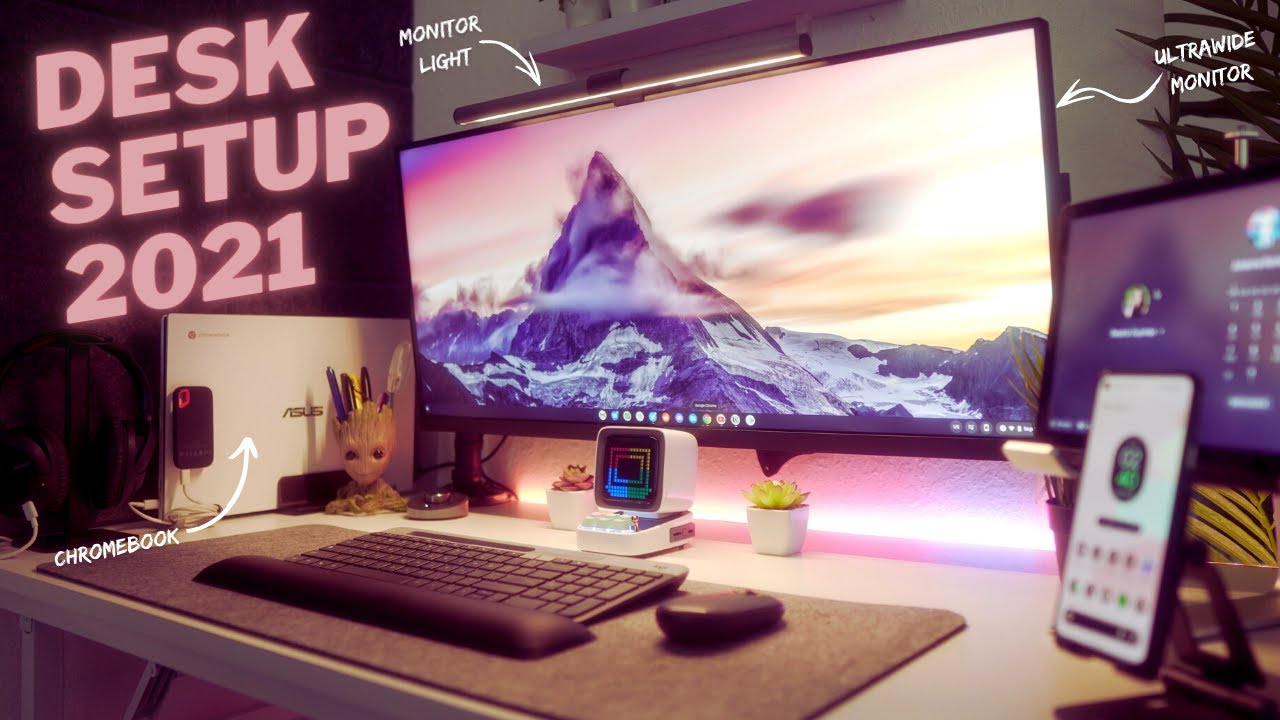This photograph showcases a detailed office workspace labeled "Desk Setup 2021." At its center is a prominent ultrawide monitor displaying a picturesque image of a snow-capped mountain peak shrouded in clouds against a vibrant sky of purples, grays, yellows, and whites. Above the monitor is a small, sleek light bar, identified by an arrow as the "monitor light." Directly in front of the monitor lies a black keyboard, complete with a cushioned wrist rest, and a black mouse, all situated on an expansive rectangular mouse pad that covers the majority of the white desk surface. Positioned to the left of the monitor is a Chromebook standing on its side, and next to it, a pencil holder shaped like a character named Gronk. On the right side of the workspace, there is a charging holder with a smartphone and a smaller monitor with a purple background behind it. Additionally, a camera is mounted on the top of the ultrawide monitor, rounding off the high-tech and meticulously arranged desk setup.